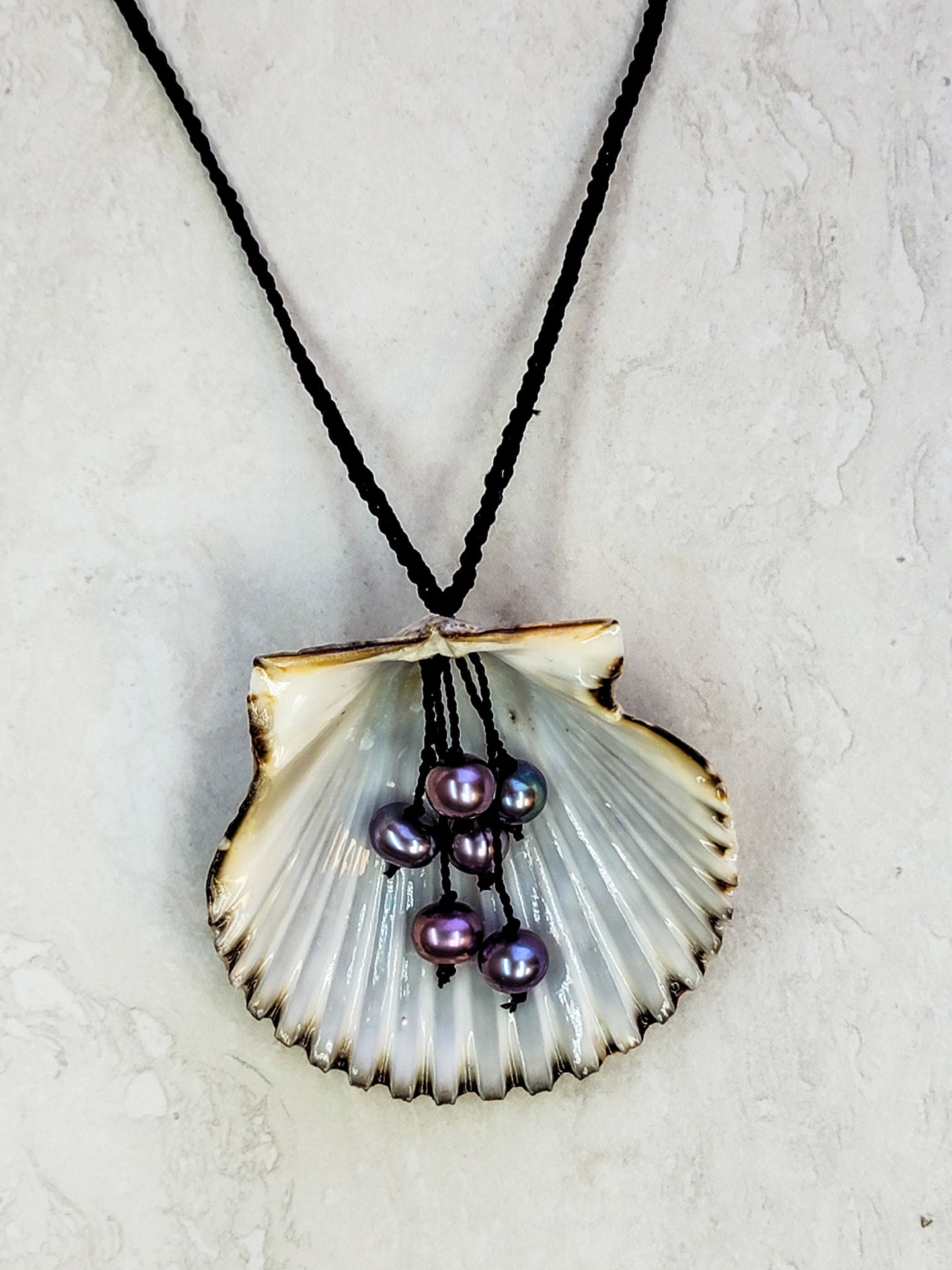The image depicts a delicate handmade necklace featuring a white clamshell pendant at the end of a black cord. The clamshell boasts a pearly-white hue with a distinctive black outline on its outer edges. The surface of the shell showcases a ripple effect, accentuating the transition from gray to white, and ultimately to black along the edge. Attached to the upper portion of the shell by black strings matching the necklace cord, are six iridescent beads that catch and reflect light, displaying shades of purple, aqua, and violet with a touch of sparkle. The necklace is elegantly presented on a white marble-like background, adding to the overall sophisticated appearance. Glares on the beads and shell highlight their glossy, polished finish.